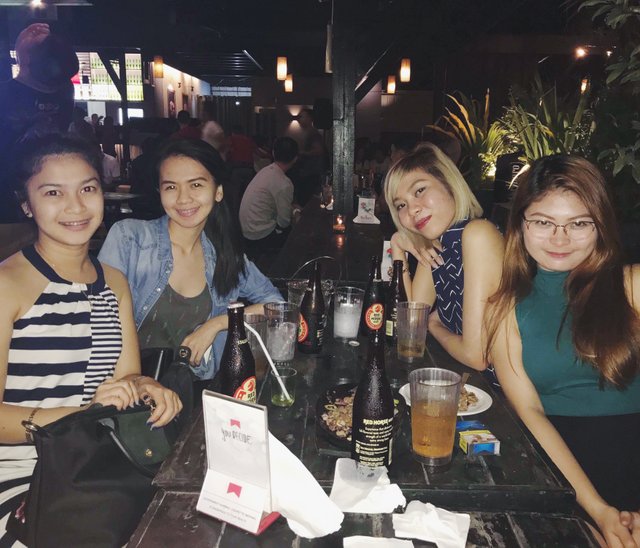In a cozy, dimly-lit restaurant bar, four young women, likely in their late teens to early twenties, are gathered around a long black table adorned with an array of drinks and light snacks. The group appears to be of Asian descent. There are two women on each side of the table, engaged in conversation and enjoying their time together. 

The woman on the far left is dressed in a navy blue and white striped tank top. Next to her, another woman sports a denim shirt over a gray tee and has long, black hair. On the opposite side of the table, one woman with short blonde hair, accessorized with a distinct blue and white shirt and bold red lipstick, sits alongside a friend with long auburn hair, glasses, and a green top.

The table is strewn with bottles of beer, glasses filled with amber and clear liquids, and a bowl of nuts. Around them, the restaurant buzzes with activity; patrons occupy similar tables, and the bar area can be seen towards the left. To the right, green plants add a touch of nature to the backdrop, complemented by lantern-like lights hanging from the ceiling, casting a soft glow. The scene is a lively mix of black, white, gray, brown, green, blue, pink, and yellow hues, capturing a vivid evening out among friends.